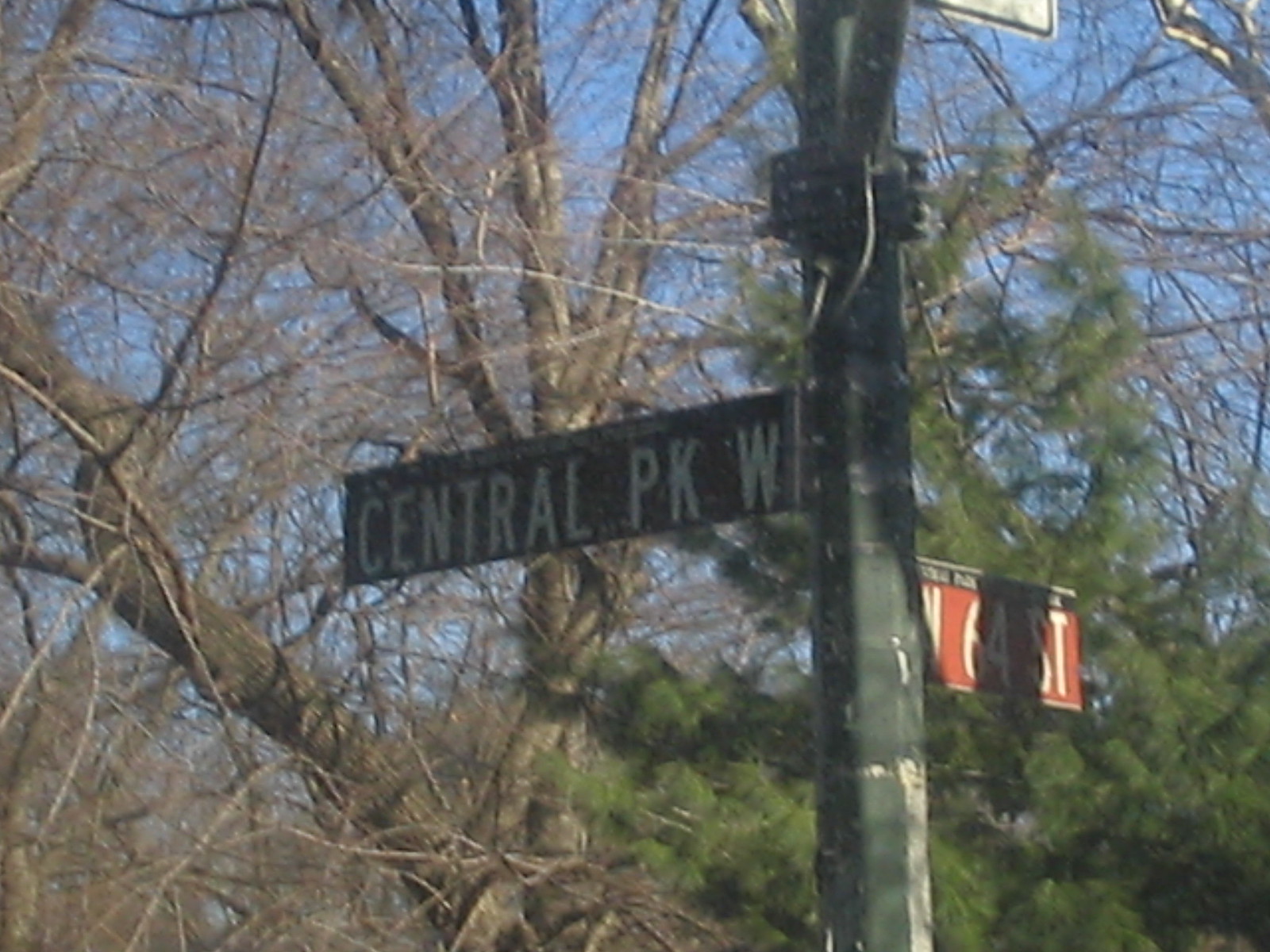The image captures a somewhat blurry, close-up view of street signs mounted on a tall, rusted, and weathered red light post, suggesting the need for a fresh coat of paint. The scene is set in New York, marked by the signs pointing to Central Park Way and West 64th Street. The Central Park Way sign is green, while the West 64th Street sign is red. The background features a vivid blue sky on a sunny day with no clouds, framed by various trees. One prominent tree with bare branches contrasts against a nearby pine tree, which is lush with needles, indicating a fall or winter setting. The photo appears to be taken from inside a moving vehicle, hence the slight blur, and features an expansive view upwards showing the sky through the bare branches.